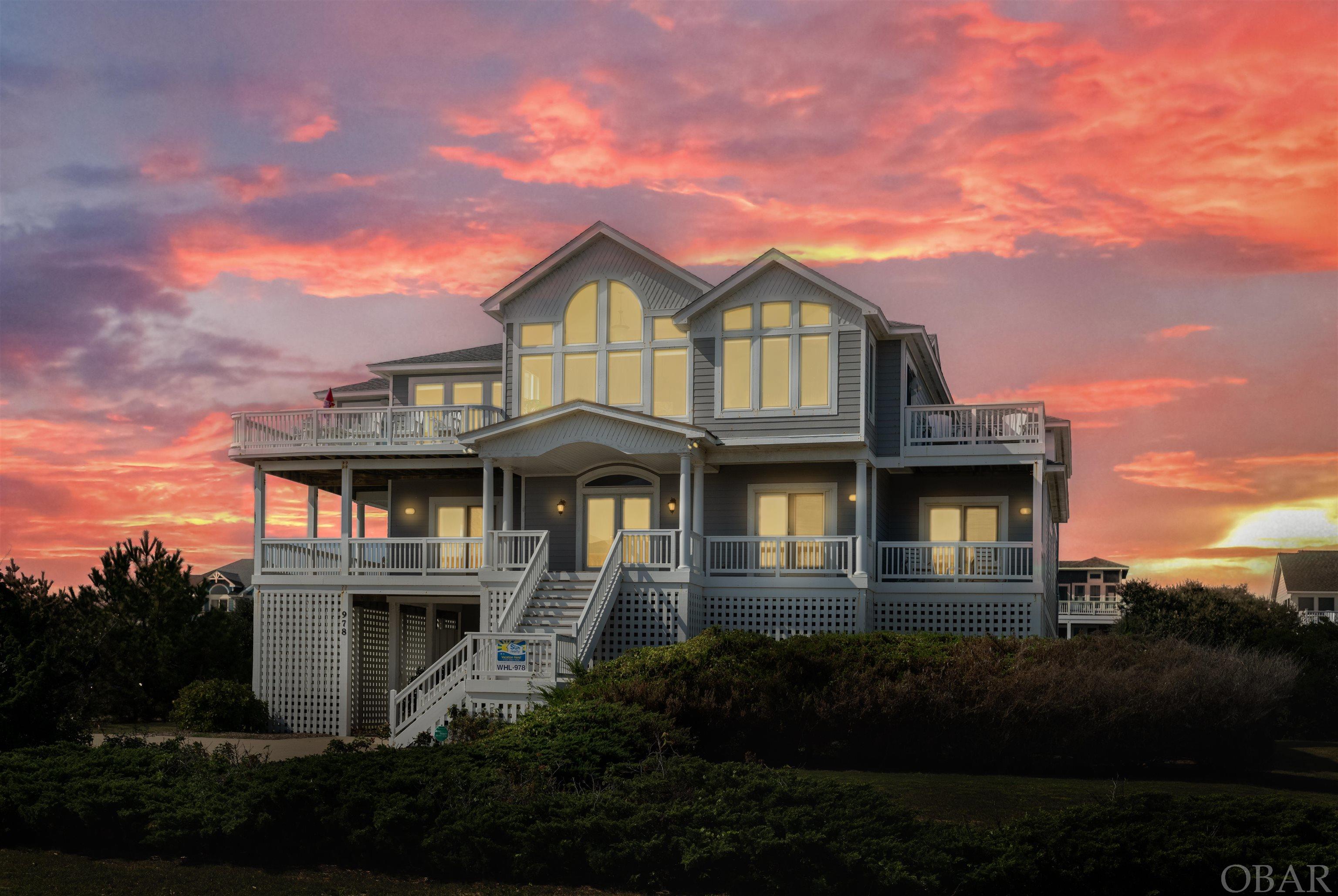The image captures a picturesque, multi-story beach house at sunset, prominently labeled "O-B-A-R" in the lower right-hand corner. The house appears to be three stories tall, constructed in a soft pastel blue or gray color with numerous floor-to-ceiling windows that glow with interior lights. It features multiple decks and patios including a wide veranda at the front and several staircases leading to different entrances. The main structure seems to sit atop a possible basement or garage level, giving it an elevated stance. Surrounding the house are lush green shrubs and grass, along with small trees, contributing to a verdant setting. The sky, filled with high clouds, reflects a breathtaking spectrum of blues, purples, oranges, reds, and yellows, typical of a sunset. Additionally, there are nearby structures visible, such as a smaller building behind and possibly another house off to the left.